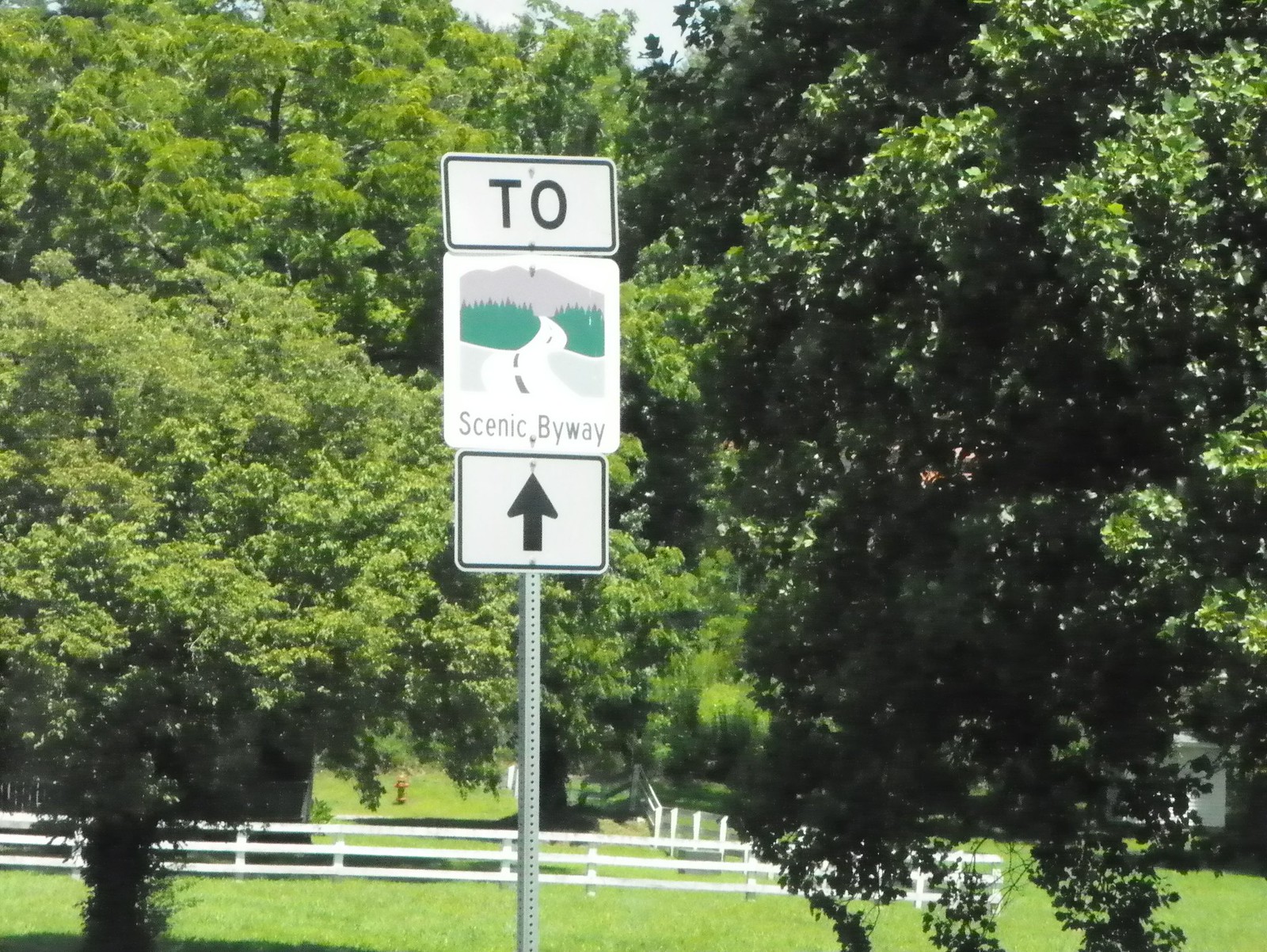This color photograph showcases a Scenic Byway street sign set against a vibrant natural backdrop. The sign, centrally positioned, stands tall on a white metal pole. The top part of the sign features black letters "T" and "O" on a white background. Below this, there is a detailed depiction of a road flanked by greenery, with a mountain in grey at the top, accompanied by the text "Scenic Byway" rendered in grey. At the bottom of the sign, a separate rectangular section with a black border contains an upward-pointing black arrow.

The background reveals a contrasting arboreal landscape. On the left side, the trees are lush and green, while on the right, the trees appear darker with only small patches of green. Above the sign, a small strip of sky is visible. Below the sign, a white fence extends through the green grass. The bottom right corner of the image hints at a possible building partially obscured by the trees and fence.